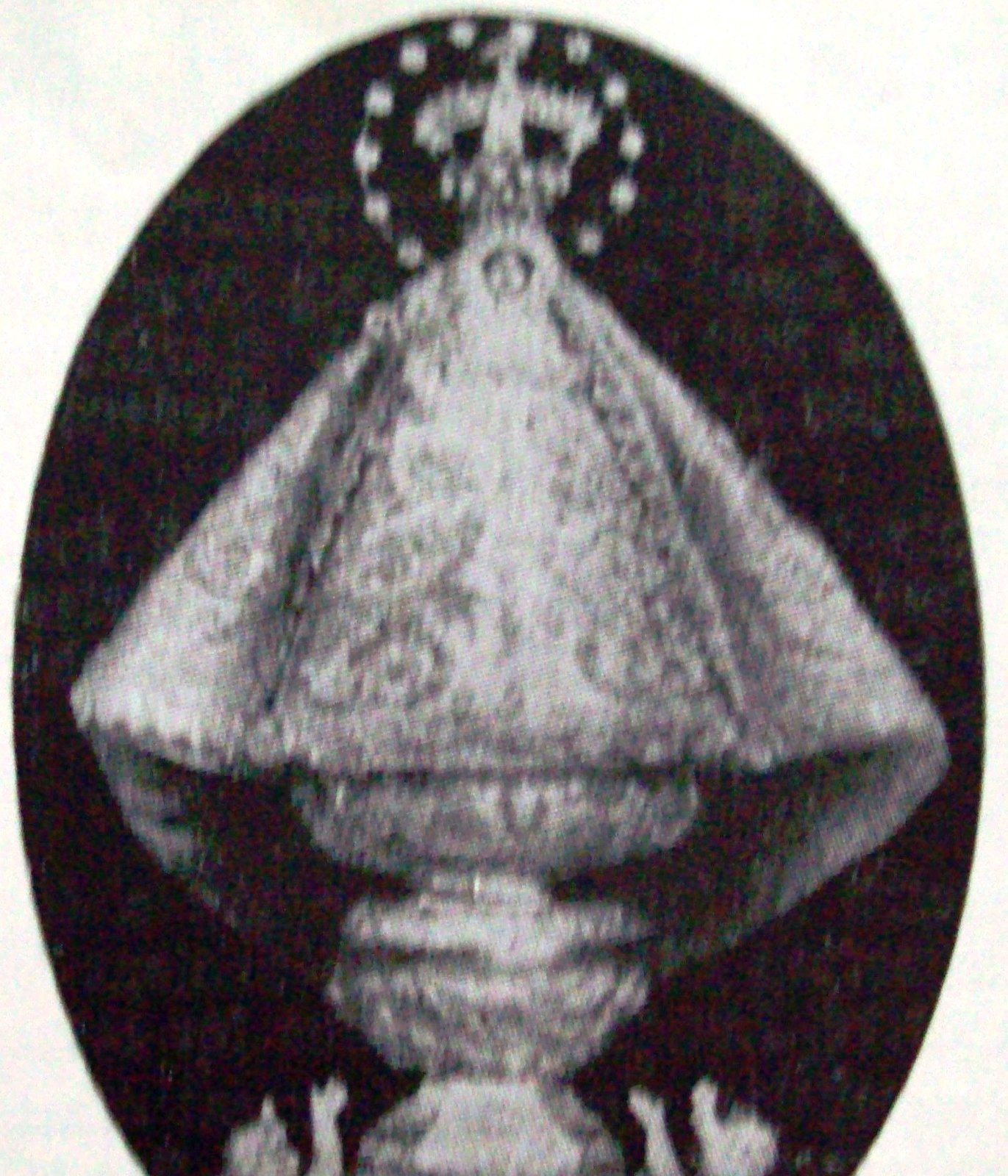The image is a black-and-white vintage photograph, portrait in orientation. It prominently features a large black ellipse with a light gray background. Inside this ellipse, there is an ornate silver relic resembling a veiled monstrance, giving the appearance of a trophy-shaped bottom draped in brocade fabric. Towering from the top of this structure appears to be a small head or portrait, resembling a queen, adorned with a crown and a circle of stars around it. This entire setup gives an impression of a grandiose, almost surreal object. At the very bottom, there are two cherubic figures or children, posed with their heads tilted upwards and arms outstretched towards the relic, as if in adoration or support. The intricate details and vintage style suggest a religious or ceremonial significance to the depicted scene.